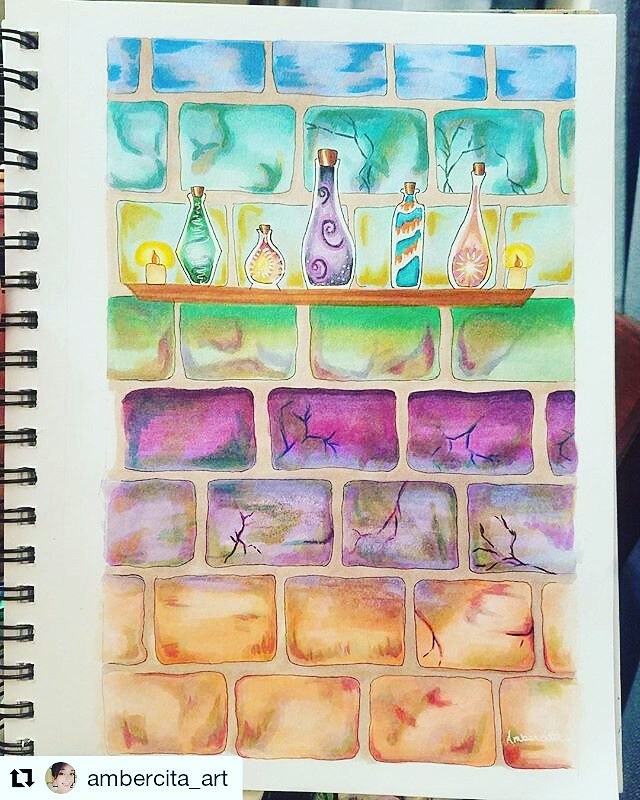This image showcases a page from a book or sketchbook, identifiable by the visible wire binding on the left side. The page is oriented in portrait mode, making it taller than it is wide. Dominating the page's design is a depiction of a wall constructed from bricks or tiles of varying colors. Around one-third of the way down the page, a small shelf is integrated into the wall, holding an assortment of items, including candles and bottles containing substances of green, purple, and yellowish hues.

The tiles themselves are arranged in distinct rows, each featuring a unique color scheme. The top row presents a mix of white and blue tiles. The subsequent row displays a combination of greenish-blue, white, and yellow tiles. Further down, the tiles begin to suggest landscape imagery. Below the landscape tiles, there is a row of purplish tiles, followed by a row of lighter purple ones. As the bricks near the bottom of the page, they progressively fade into different colors, creating a gradient effect that enhances the visual depth and interest of the composition.